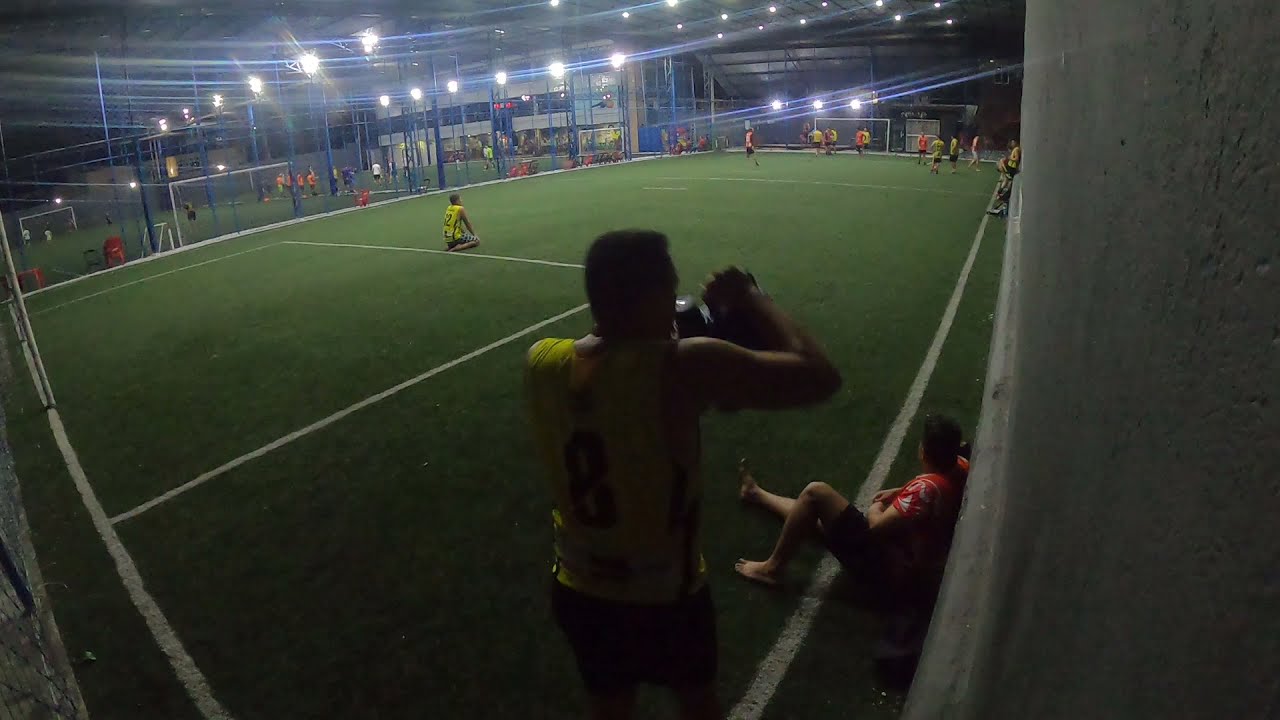This image captures an indoor soccer game played on a nighttime, green turf field marked with white lines. The photo is taken from one corner, offering a broad diagonal view of the entire field. In the foreground, a man in a yellow jersey kneels, while another in a red jersey sits on the sideline. Most players, wearing either yellow or red jerseys, are seen in the distance. The field is bordered by tall floodlights and includes see-through partitions on the left side, suggesting there's another adjacent field. A gray wall is located in the right corner, and in the far background, a field house with windows and a metal roof is visible. Some chairs are scattered near the sidelines, and the goals are positioned at the left and far ends of the field.